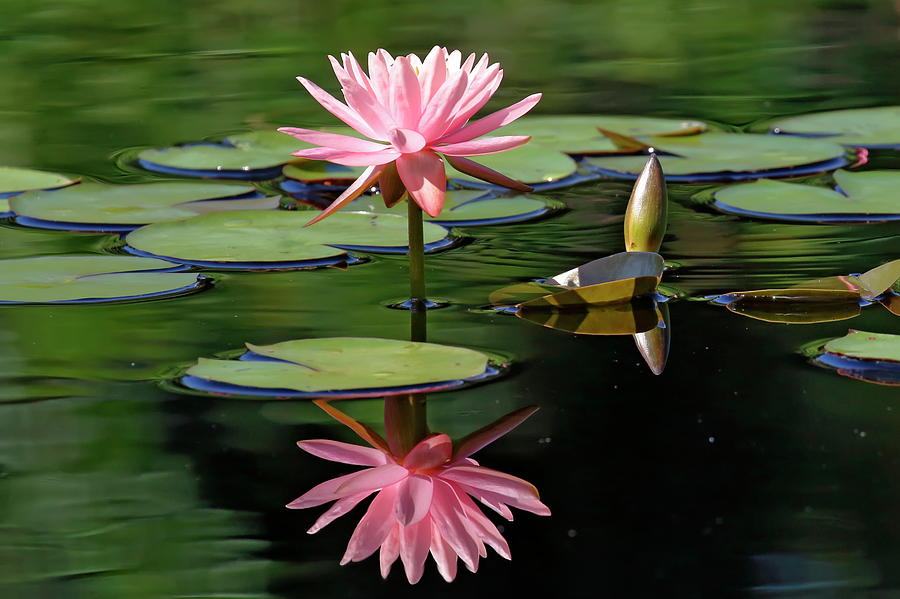This rectangular image features a tranquil pond adorned with a spread of large, green lily pads floating on its surface. In the center of the scene, a striking pink water lily, with its petals splayed out like a starburst, rises gracefully from the water on a thick, prominent stem. The water around the lily pads exhibits a play of light and dark green hues, likely reflecting the surrounding canopy of trees and shrubbery, creating a dynamic, rippled effect. The composition captures a vivid reflection of the pink flower on the water's surface, creating a mirage-like image where the flower appears to exist both above and below the waterline. The detailed interplay of natural elements and reflections imbues the scene with a serene and picturesque quality.